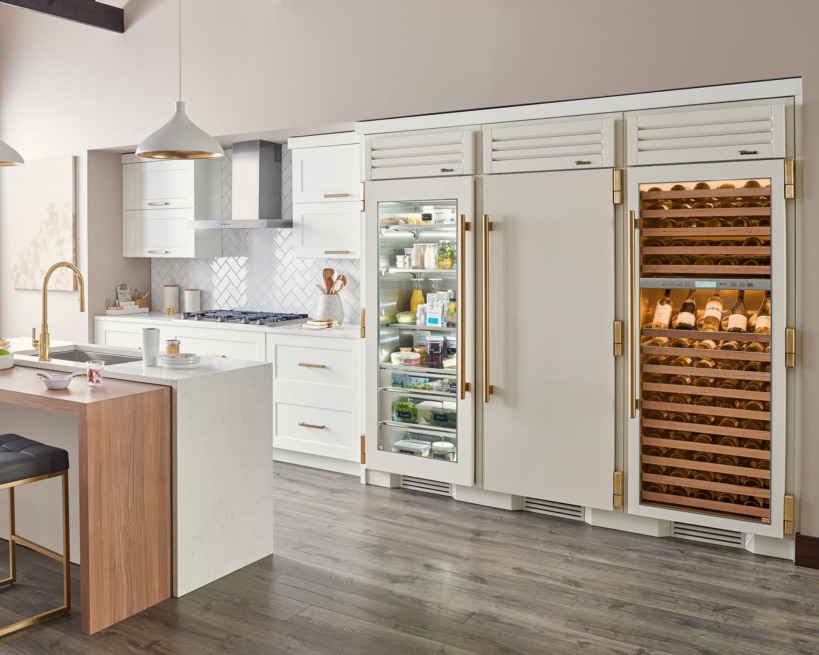The photograph showcases a luxurious, modern kitchen bathed in both artificial and natural light. The kitchen features grayish brown wood plank flooring that complements the light gray painted walls. On the bottom left corner, there's a pristine white kitchen island equipped with a deep farmhouse sink, highlighted by its large, curved golden faucet. Adjacent to the back of the island is a small, thin brown wooden bar table, accommodating a gold-framed, black-cushioned chair. The tabletop holds a white dish with a matching spoon, a clear glass adorned with floral patterns, and a white pot containing a vibrant yellow flower.

To the right of the scene, there's a sophisticated wine cooler with illuminated wooden racks filled with bottles. Next to it stands a sleek professional-style refrigerator ensemble, including a floor-to-ceiling wine fridge, a closed refrigerator, and a glass-door refrigerator, all with gold handles and trims. The kitchen also boasts a white countertop on the left, framed by medium brown wood paneling, and features white cabinets adorned with gold hardware. A herringbone white tile backsplash adds texture behind the gas cooktop and stove, complemented by an overhead air blower. This gourmet kitchen is complete with stylish and functional elements ideal for both cooking and casual dining.